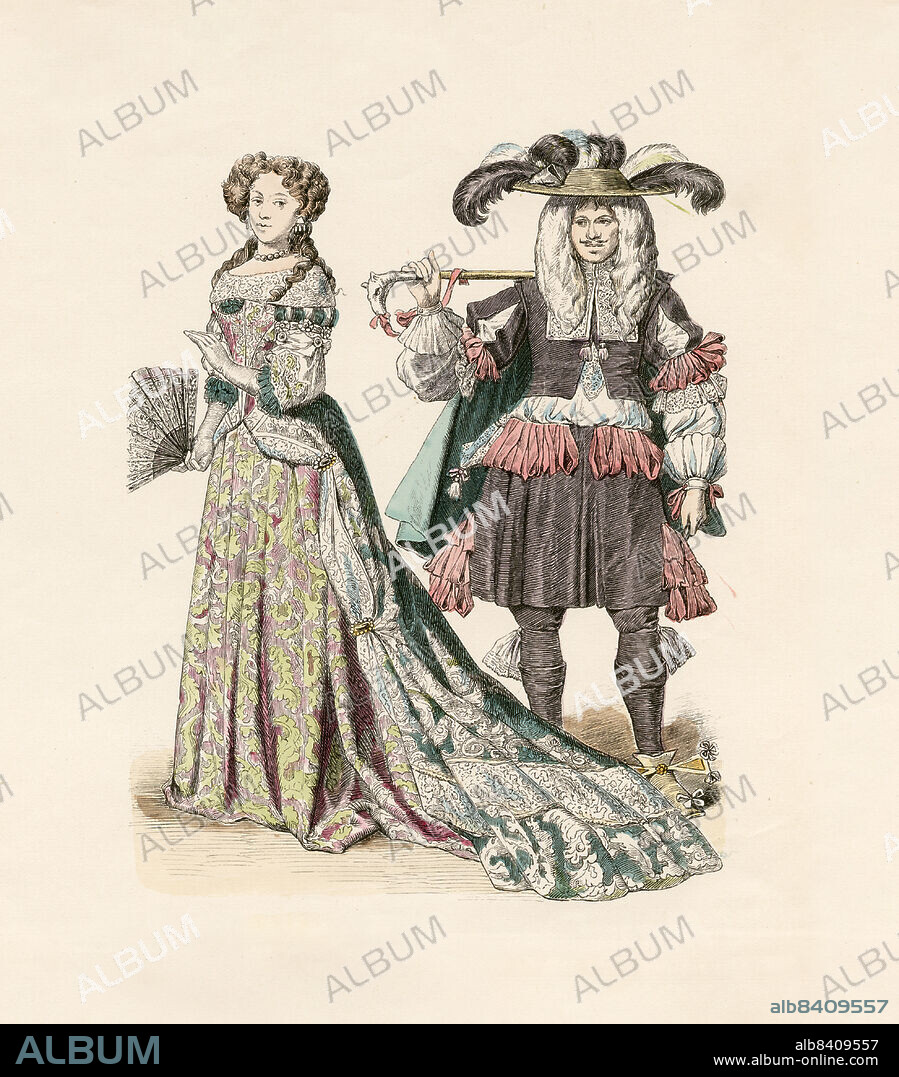This digital or colored pencil rendering depicts two elegantly dressed individuals from the medieval or early modern era, set against a beige-pink background. The image features a repetitive watermark, "ALBUM," in grey, cascading across the background. At the bottom of the image, a black rectangle contains the word "ALBUM" in cyan letters, alongside a website URL: www.album-online.com. To the right, in white text, are the characters "ALB8409557," repeated directly above in bluish-green text.

The woman on the left, possibly Maria Anna of Bavaria as the crown princess of France, is dressed in a lavish court dress. Her shoulder-length, curly brown hair with orange accents frames her light-completed face. She wears a pearl necklace and grey earrings. Her attire is meticulously detailed: a two-piece dress where the upper part is grey with greenish-blue accents at the sleeve ends, and hints of purple just below her chest. The lower part features a green and pink floral pattern. Cascading behind her is another section of her dress in grey-white with greenish-blue accents, adding to the ensemble’s grandeur. She holds a delicate hand fan in her left hand, and wears white-grey gloves.

Standing beside her is a young dandy from the same period, dressed in equally intricate attire. He dons a flat, feathered cap and has long grey hair that falls just past his shoulders. In his left hand, he holds a gold cane topped with a dragon or dog’s head, complete with red feather embellishments. His outfit consists of a puffed brown tunic with red frilled edges, a white undershirt with visible embroidered collar, and a greenish-blue cape. The tunic's sleeves are adorned with red puffs and an embroidered white pattern just before his hands. His leggings are brown, complemented by light brown shoes that tie around his feet.

In summary, this detailed rendering captures the ornate fashion and elegant demeanor of these two historical figures against a softly tinted background, emphasizing the period's grandeur and intricate clothing designs.